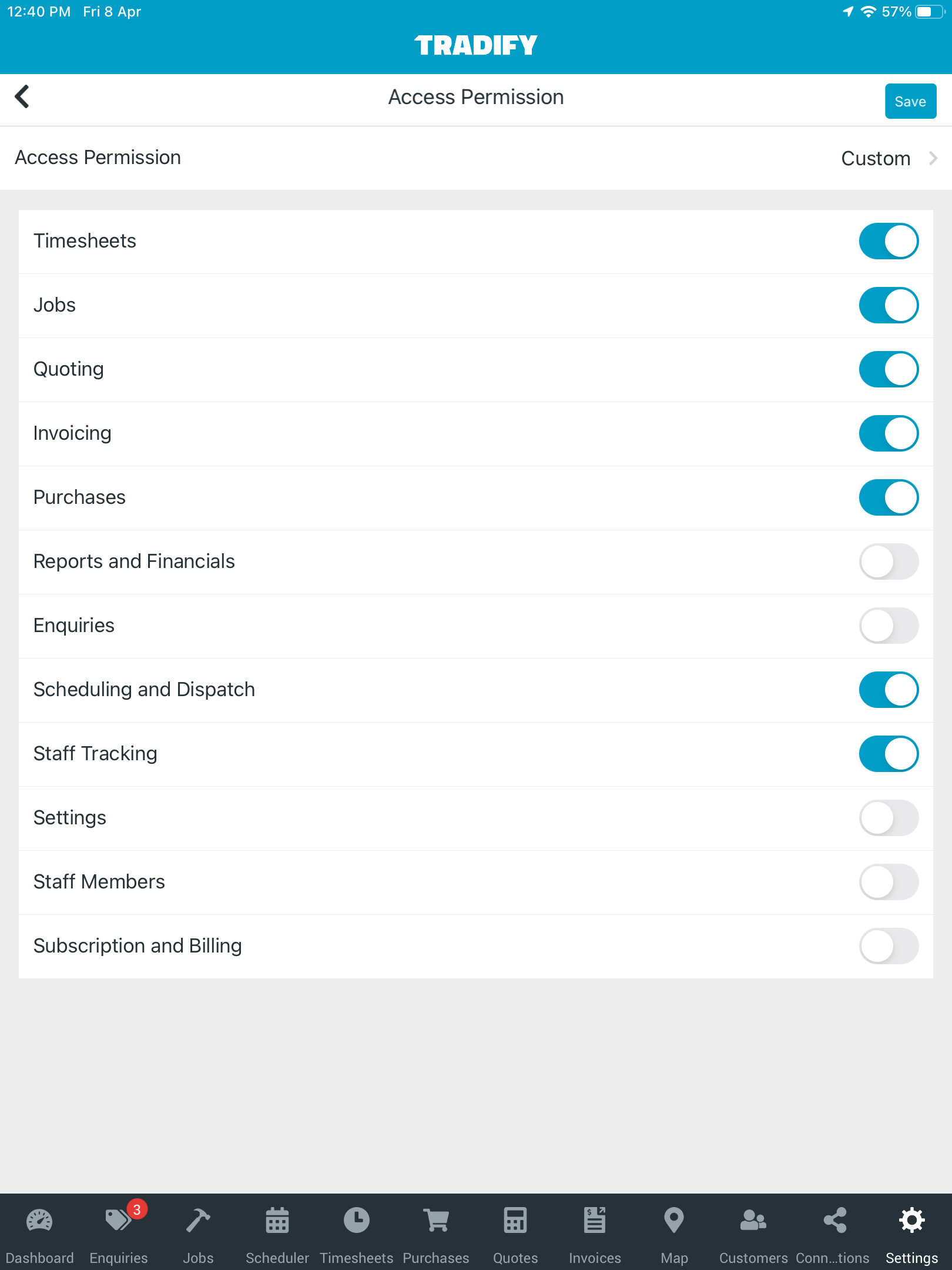**Detailed Descriptive Caption:**

The image is a screenshot of a tablet displaying an access permission settings page, formatted in portrait rectangle. The screen is dominated by a light to medium blue header at the top with white text. In the upper left corner, small text reads "12:40 PM, FRI 8 APR" with 'PM', 'FRI', and 'APR' capitalized. Centered in big, bold, all-caps font is the word "TRADIFY." In the upper right corner are several icons: an upward-pointing thick arrow, a full-strength internet signal icon (represented by ascending semi-circles), the numbers "57%," and a battery icon indicating 57% charge.

Below the blue header, the main section has a white background. Centered at the top, it states "Access Permission." To the far right is a 'Save' button, a medium blue rectangular button with rounded corners and white 'SAVE' text. To the left of "Access Permission," there's a left-pointing arrowhead.

Below this header section, another section is underlined in white. On the left, it again says "Access Permission;" on the right, it says "Custom." The background here is light gray, with a white background square area showing a list of 12 settings. These settings are left-justified, each separated by thin gray lines, and have toggle switches on the right.

The toggles are oval, with a white button that slides. When on (button to the right), the background is medium blue; when off (button to the left), the background is light gray. The first five settings ("Timesheets," "Jobs," "Quoting," "Invoicing," "Purchases") are toggled on. The next three settings ("Reports and Financials," "Inquiries") are toggled off. The following two settings ("Scheduling and Dispatch," "Staff Tracking") are toggled on. The last three settings ("Settings," "Staff Members," "Subscription Billing") are toggled off.

Below this white section is a substantial light gray field, leading to the footer. The footer background is black and contains 12 icons with labels beneath them. All icons and labels are light gray, except for the far-right one which is highlighted indicating selection. This icon has a gear above the word "Settings." The far-left icon represents a dashboard and has an odometer icon above it. The second icon represents inquiries, depicted with ticket icons and a red circle with a white "3," indicating three unread inquiries. The third icon is labeled "Jobs" with a gray hammer icon above it. This pattern continues across the footer with varied icons and labels for different functions.